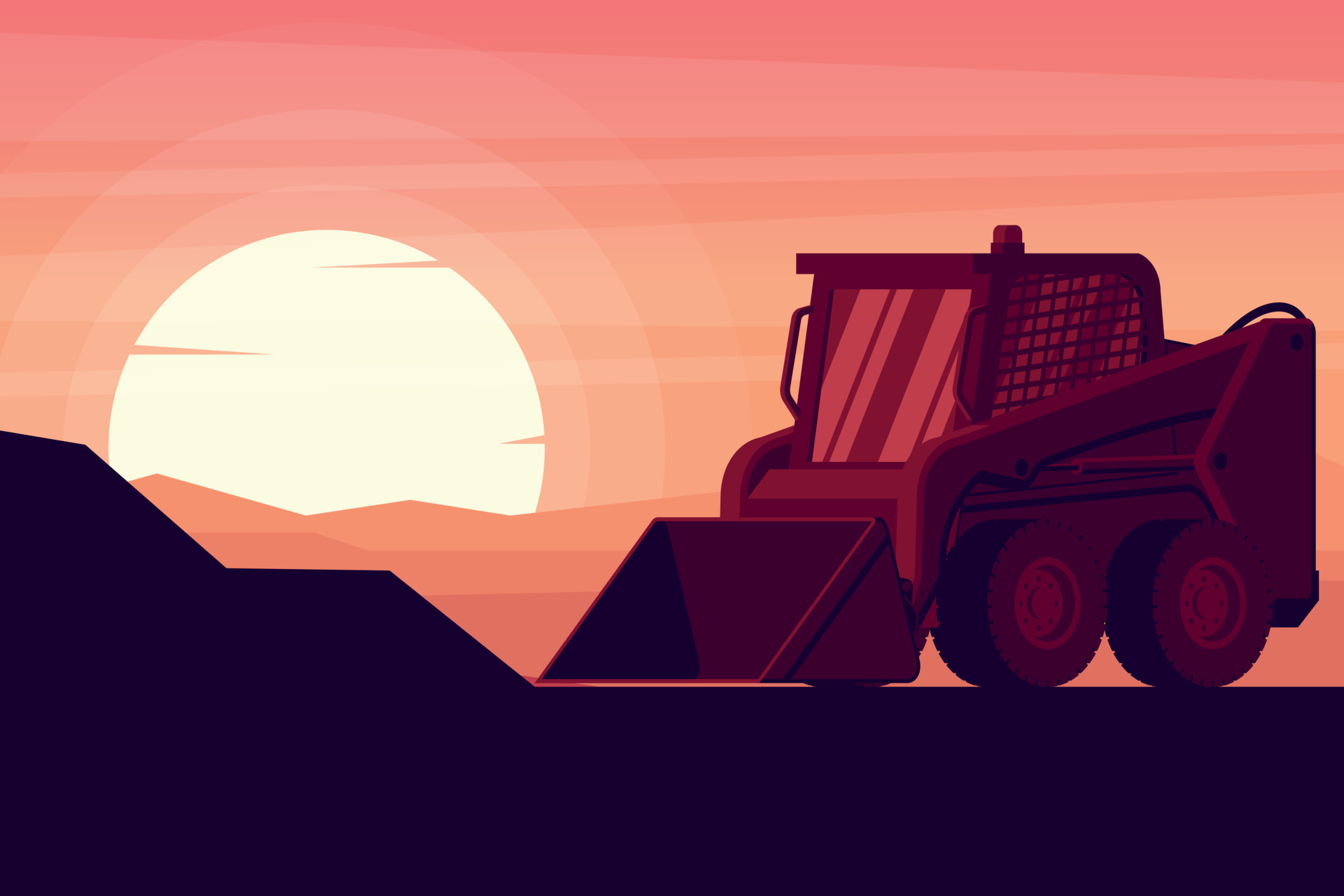This is an AI-generated, minimalistic 2D illustration depicting a front loader, sometimes referred to as a skid-steer or bobcat, engaged in a construction task. The front loader, characterized by its large metal bucket connected to two hydraulic arms on each side, appears to be navigating a step-like gravel pile. The vehicle exhibits unique design choices, including an unconventional window and protective metal grate mesh on the right side, and possesses two large wheels with heavy treads on each side. The cockpit, where the driver sits, is shielded by a light on the roof and dark hydraulic lines at the back. 

In the background, a massive, unrealistic sun illuminates the scene with its glowing yellow, pink, and orange hues, suggesting it is either sunrise or sunset. The sky is streaked with white lines resembling clouds. The landscape features a silhouetted row of pinkish hills providing a stark contrast against the somewhat darkened foreground. Overall, the minimalist rendering emphasizes large, single-color shapes without intricate textures or shadows, giving it a flat, almost surreal appearance.